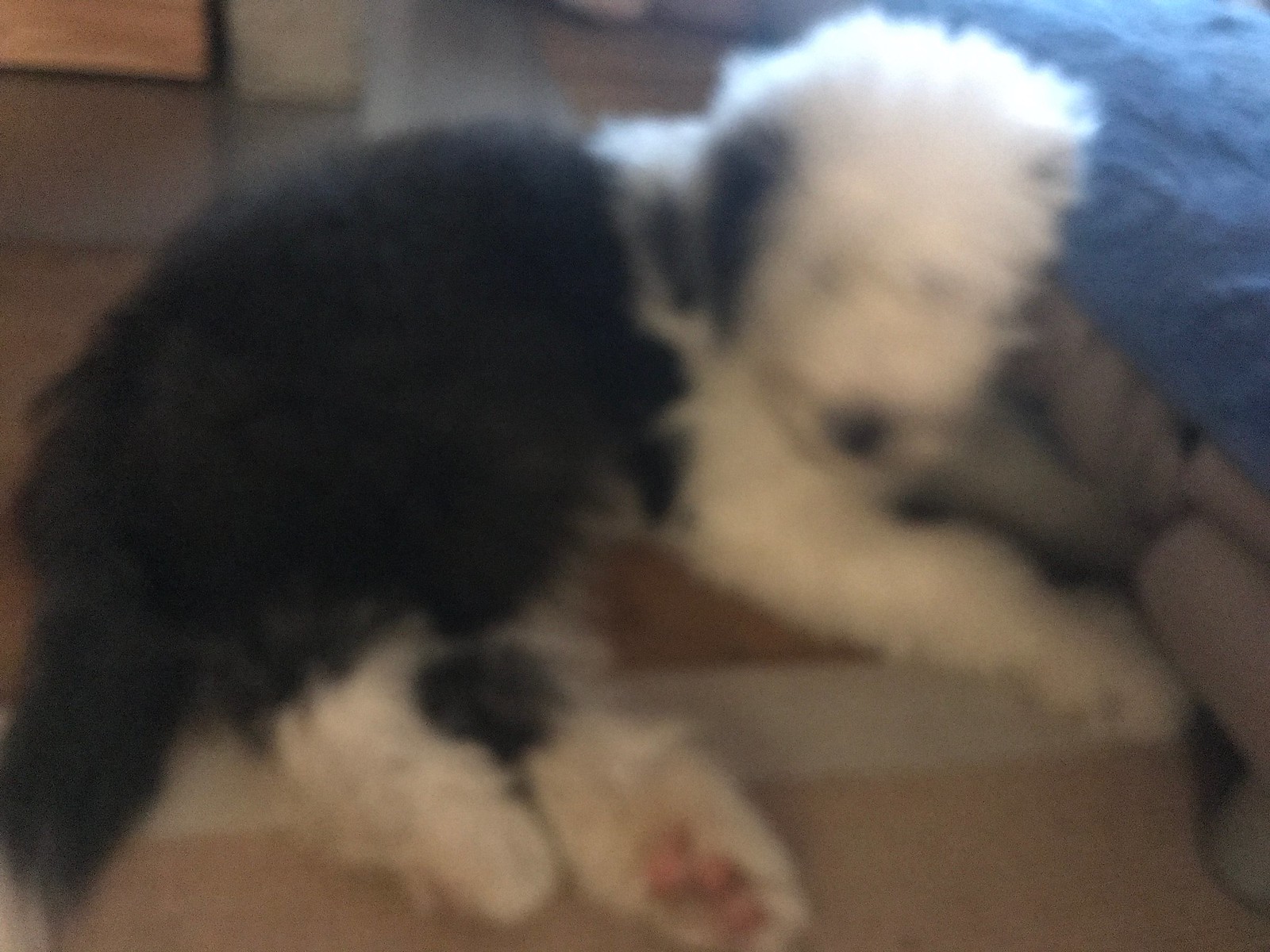In the image, a very blurry dog is lying on its side on the floor. The dog has a fluffy white head with a shorter snout and a black nose, giving it a distinctive appearance. Its front right paw is stretched out while its rear paws are curled up underneath its body. Notably, all of its paws are white. The left half of the dog's back is a darker color, almost black, and it has a long black tail that extends out behind it.

The flooring beneath the dog features a gray strip, partially obscuring the floor's texture. The dog appears to be next to a piece of furniture on the right side of the image, possibly a bed, which is covered in blue fabric. In the top left-hand corner, the bottom of a wooden box is visible, along with a grayish container situated next to it.